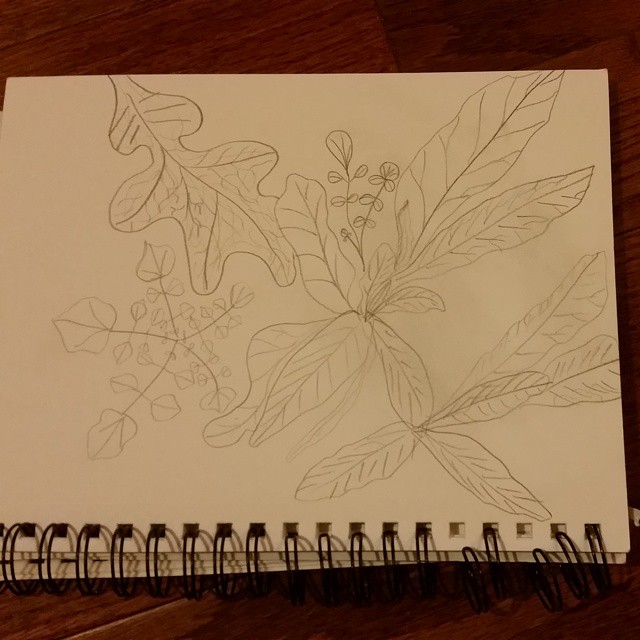The image showcases a detailed pencil sketch on a white piece of paper that is still attached to a black spiral-bound notebook. The notebook is positioned with the spiral binding at the bottom, lying open on a dark brown, wood-paneled floor. The sketch itself features a variety of leaves and a prominent central flower. The larger leaf in the background has swirling, curvy edges with visible veining. The central flower boasts long, thin petals that extend outward and taper at the tips. Surrounding this focal flower, the sketch includes approximately five or six different types of leaves: some are large and singular, others are composed of small leaves branching out from slender stems. There are also unique formations, like clusters of four skinny leaves connected at a central point, and larger leaves with smaller offshoots. Despite the detailed renderings, the drawing maintains a simple, uncolored aesthetic with significant negative space, giving it an unfinished yet organic feel.